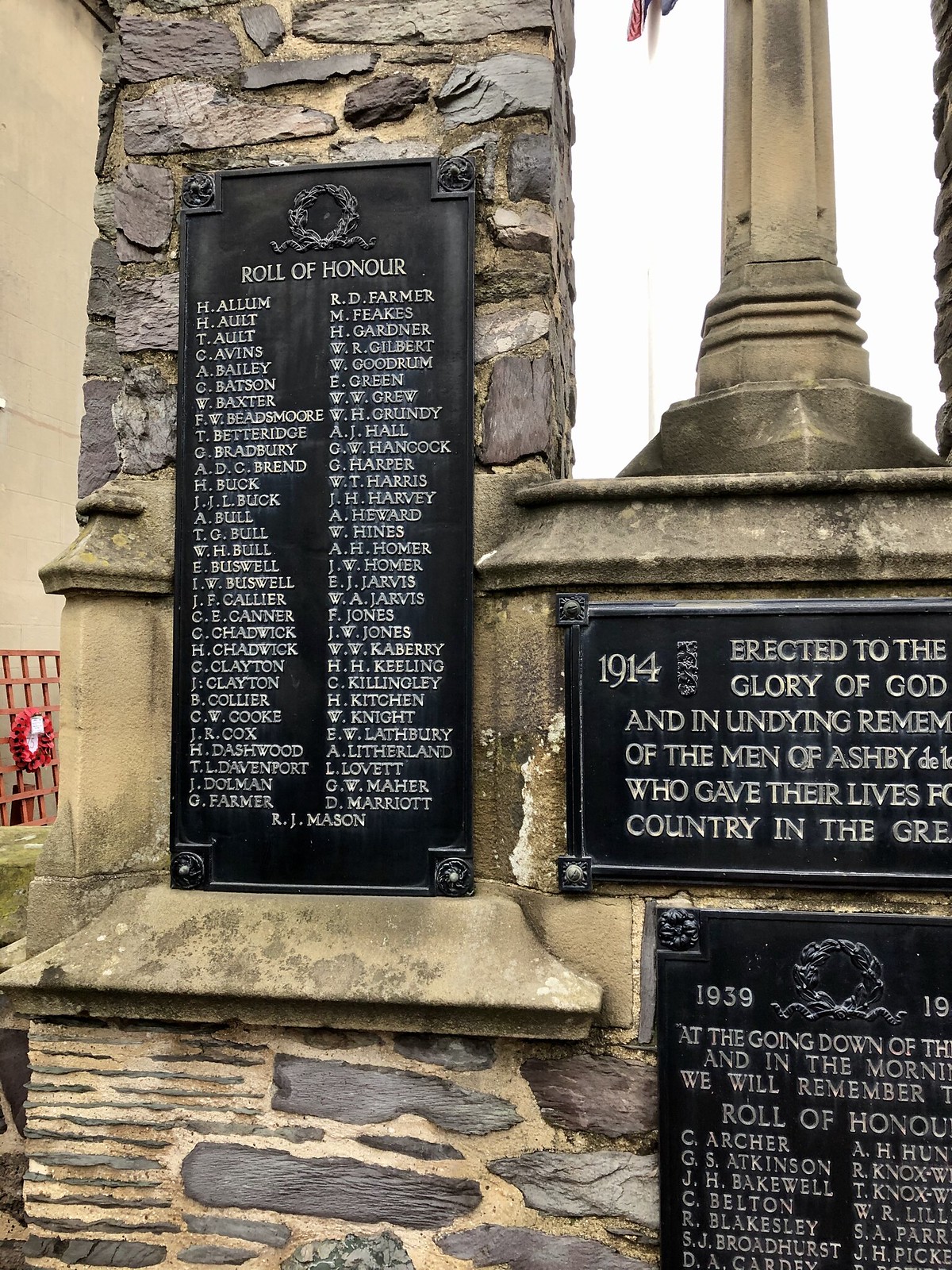This close-up photograph captures a historic stone monument dedicated to the fallen soldiers of Ashby, England, from the years encompassing 1914 to 1939. The monument showcases an aged and partially weathered black plaque bearing the inscription "Roll of Honor," and behind this is a large stone wall constructed with stone and mortar. Detailed engravings on the plaque list approximately a hundred names of the men who gave their lives. Not far from the stone wall, there's an obelisk with the dates 1914 and 1939 engraved on it, flanking the plaque. Below the obelisk, the inscription reads, "Erected to the Glory of God and in Undying Remembrance of the Men of Ashby Who Gave Their Lives for Their Country." Despite its weathered state, which includes some dirt and aging cement, the monument's solemn message remains clear and impactful.